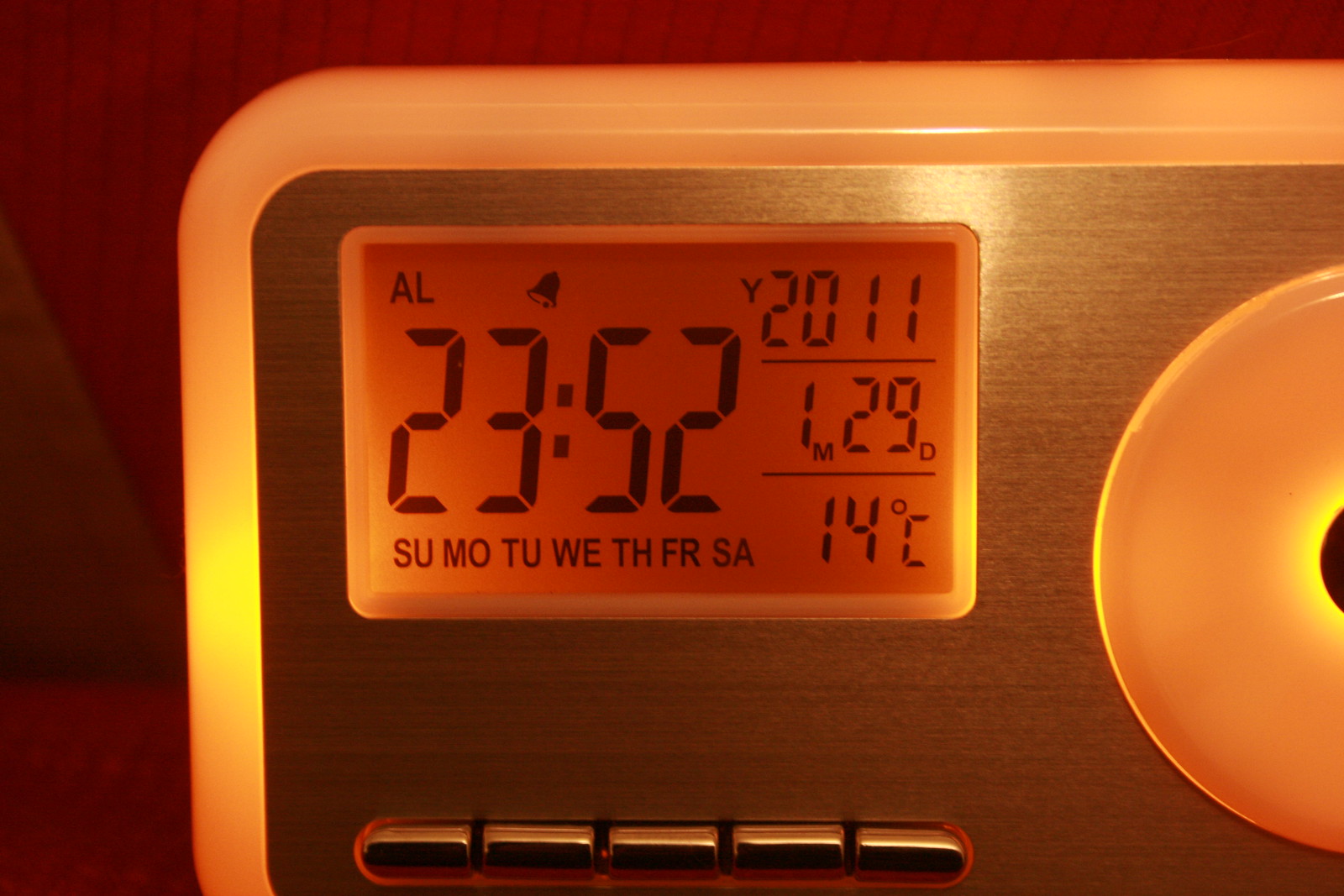The image shows a close-up of a modern clock with a brushed stainless steel face and white plastic rim, which is partially illuminated in a yellow-orange hue from the inside. The clock has a digital rectangular screen backlit in orange, displaying the current time in military format as 23:52 (11:52 PM). Above the screen, an "AL" symbol alongside a bell icon indicates that the alarm is set. The screen also shows the year as 2011, the date as January 29th, and the temperature reading of 14 degrees Celsius. At the bottom of the screen, the days of the week are outlined. On the clock's top left, there are five silver buttons, while a round, semi-visible white plastic component to the bottom left, likely a speaker, is also illuminated in orange with a central black element. The clock's design, which incorporates both brushed metal and illuminated plastic, offers a visually striking appearance reminiscent of an old jukebox. The background features a wood-like finish, adding to the overall aesthetic.